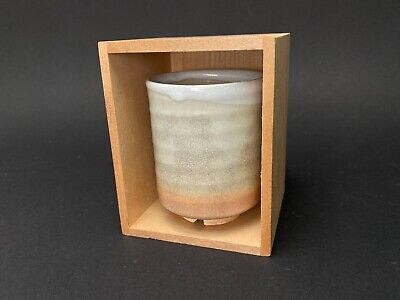The photograph showcases a scene with a completely gray background, devoid of any additional elements. At the center of the image sits a small, light brown wooden box, slightly angled to the left, which provides a clear view of its contents. The front of the box is open, revealing a handmade ceramic mug inside. The mug nearly fills the entire space of the box, with just a little room at the top and almost touching the sides. The mug's glazing features a gradient of neutral colors: the top has a thin ring of white, followed by a grayish-brown band, then a beige section, and finally, a reddish color at the base. The craftsmanship of the mug is evident from the grooves and textures, indicating it was carefully hand-thrown, making it an artful display within the wooden container against the stark gray backdrop.